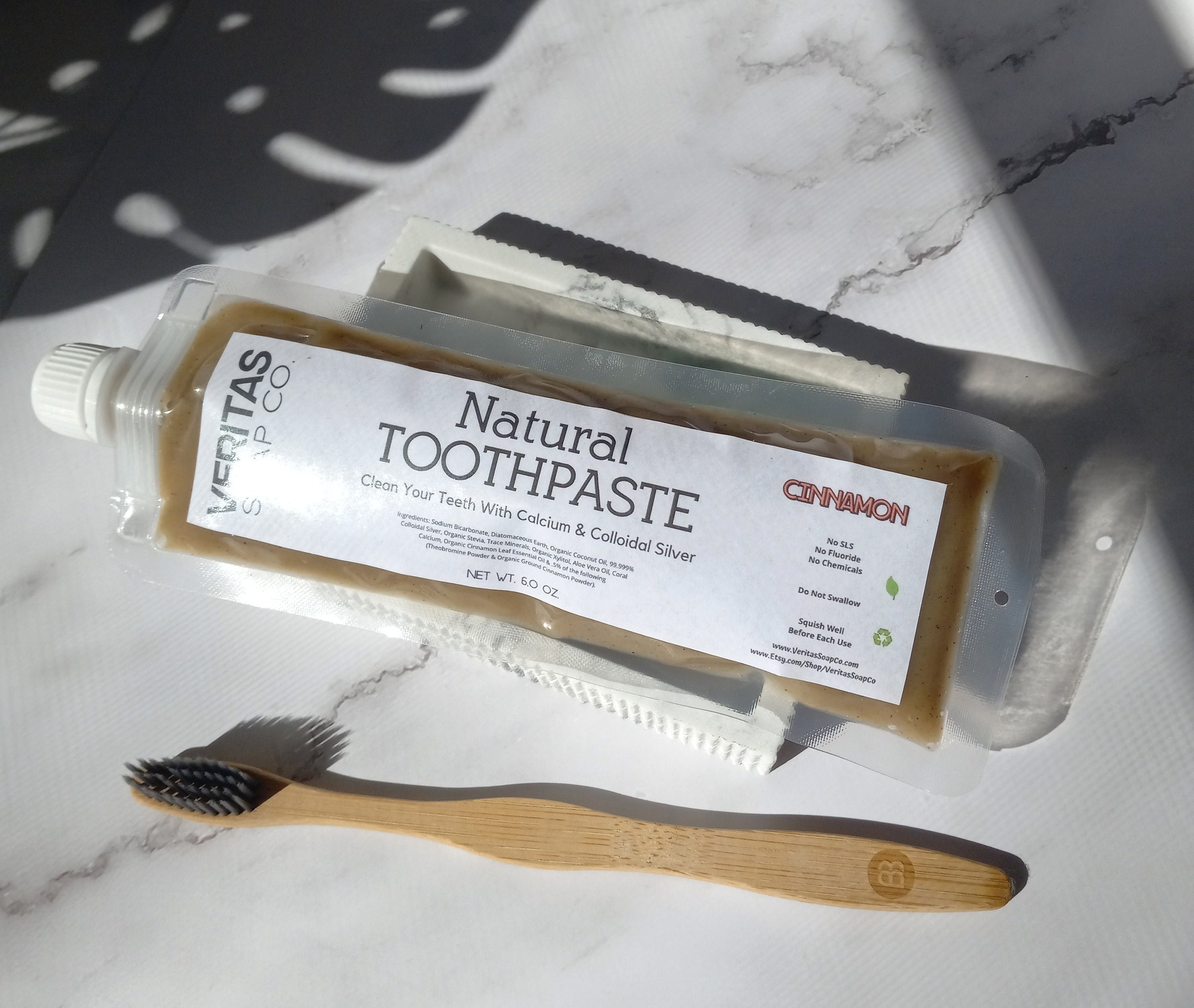The image depicts a tube of "natural toothpaste" and a toothbrush, set against a white marble surface. The toothpaste is in a transparent container with a white cap and features a white label with the brand name "VERITAS" written vertically on the left side. The label reads "natural toothpaste, clean your teeth with calcium and colloidal silver," along with the flavor designation "cinnamon" on the top right. The toothpaste itself is a brown paste, and the tube's net weight is listed as six ounces. Positioned next to the tube is a toothbrush with a wooden handle and dark gray bristles. Both the toothpaste and the toothbrush are angled towards the upper left, resting on a marble tray, with part of the blurred marble countertop visible in the background.